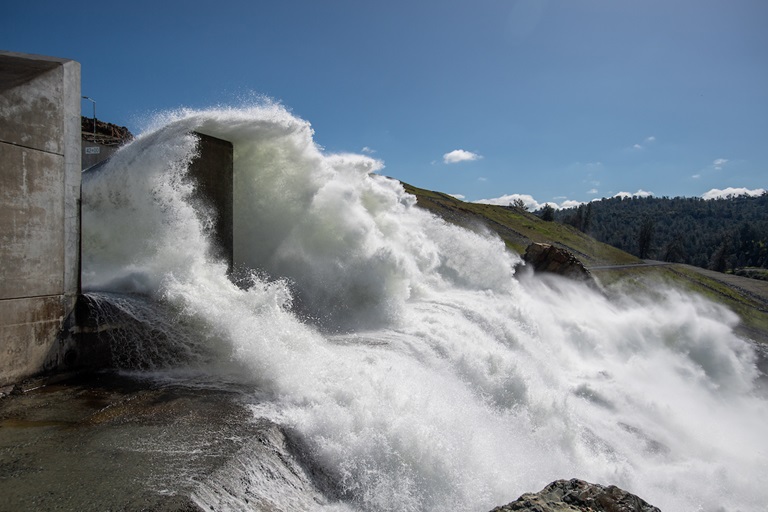The photograph captures a powerful scene of a bustling dam, constructed from dark grey concrete. To the left, portions of the dam are visible, emphasizing its robust structure. The central focus is on the intense, white, foamy water cascading forcefully over the top and descending like a waterfall, maintaining a vigorous descent towards the right side of the image. The dam integrates into the natural scenery with a grassy hill in the mid-background, which appears to be a blend of brownish-green hues and industrial patches. Big rocks jut prominently amid the surging water, adding to the dramatic visual. In the distant background, a tranquil forest rises along the horizon, predominantly composed of pine trees, under a clear blue sky adorned with soft, fluffy white clouds. The overall scene portrays a mix of mechanical might and natural beauty, emanating energy and dynamic motion that almost lets you hear the roaring water.